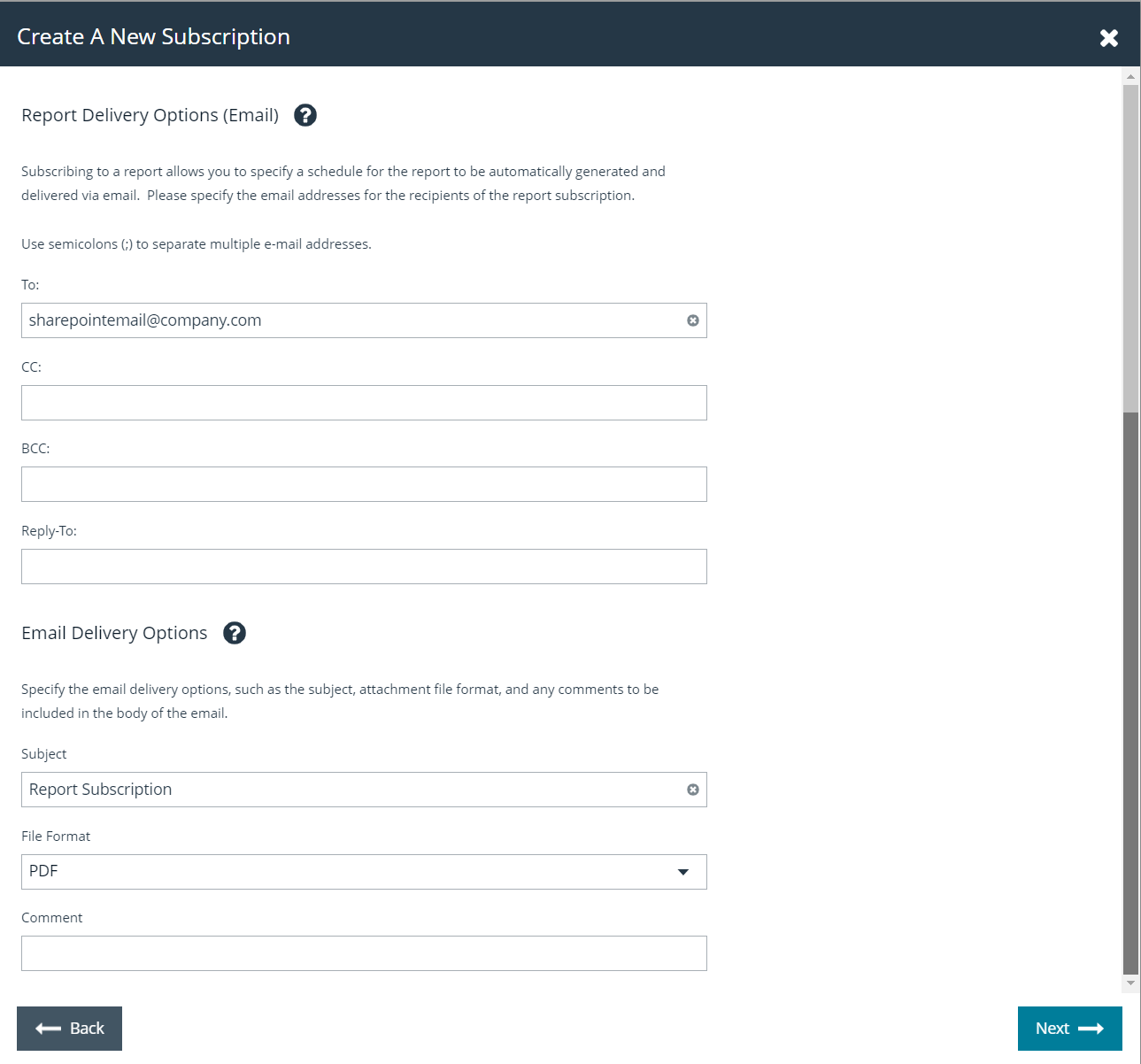The screenshot depicts a user interface for creating a new subscription. The layout features a clean white background with a navy blue header bar at the top, where "Create a New Subscription" is inscribed in white letters. On the top right side of the header is a small white "X" for closing the window. Running down the right side of the page is a vertical scroll bar, indicating that the page content can be scrolled.

Directly below the header, central to the top section of the page, is the heading "Report Delivery Options (Email)" next to a black circle containing a white question mark, likely serving as a help icon. Below this heading, there is a brief paragraph containing details that are too small to discern in the screenshot.

The page contains four horizontal input fields labeled "To," "CC," "BCC," "Reply," and an unspecified text following "Reply." Each of these fields has a corresponding box to type information. A similar heading style and help icon appear again with the title "Email Delivery Options" followed by another short paragraph. 

Further down, three additional rectangular input fields are labeled "Subject," "File Format," and "Content," each with its respective text box.

At the bottom of the page is a navigation section, featuring a black rectangular button labeled "Back" on the left and a blue rectangular button labeled "Next" on the right.